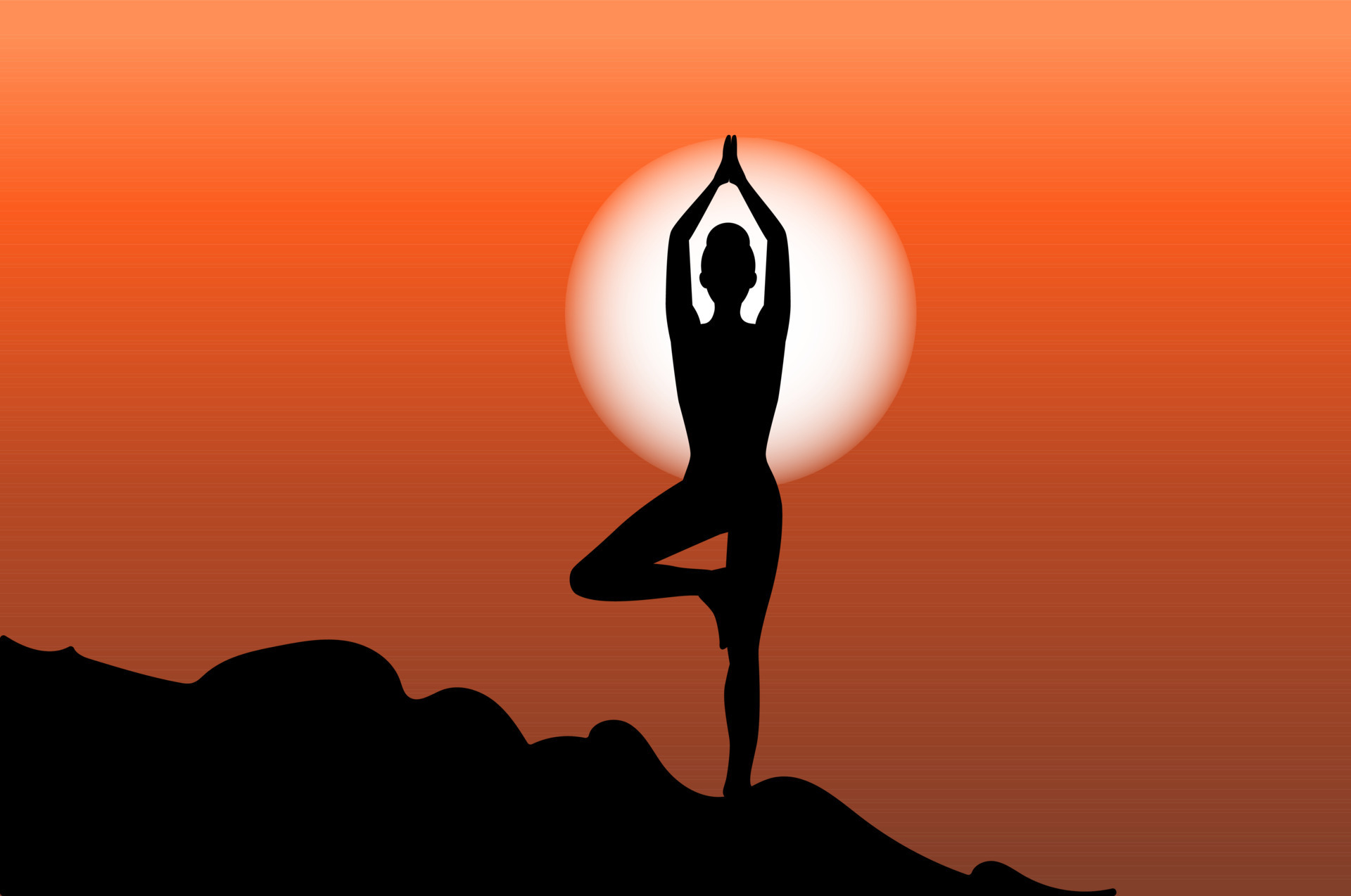The image depicts a serene and minimalist scene of a woman performing a yoga pose against a vibrant sunset backdrop. The dominant colors are shades of orange and red, with a gradient effect that darkens as it moves downward. Central to the image is a plain white orb representing the sun, positioned directly behind the woman's silhouette. This silhouette is entirely black, offering stark contrast. The woman has her hair in a bun and stands gracefully on one leg, with her other leg bent and her foot placed flat against her inner thigh. Her arms are extended upward, hands pressed together in a classic yoga gesture. She stands on a rocky slope, which also appears as a black silhouette, effectively grounding the scene. The overall composition emphasizes tranquility and balance, captured in this striking, stylized depiction of sunset yoga.